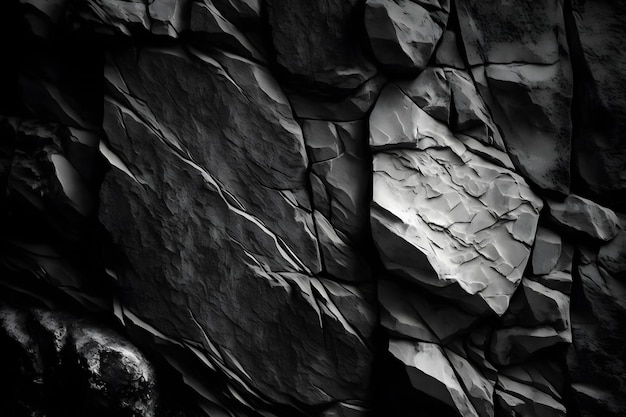The image appears to be a computer-generated 3D graphic resembling a rugged stone or rock face. The entire scene is rendered in varying shades of gray, black, and white. The left side of the image is predominantly dark, almost completely black, with some subtle highlights that hint at protruding areas of the rock. As you move to the right, the stone gradually lightens, revealing intricate details of the textured surface. These details include cracks, ridges, and bumpy areas that give the rock its rough appearance. About halfway across the image, a particularly light gray section stands out prominently, illuminated as if by a light source coming from the right. This brighter area accentuates the natural indentations and peaks of the rock surface, creating a stark contrast with the darker sections. The brightness peaks near the right end before it begins to dim slightly again, maintaining the highly textured, craggy look throughout.